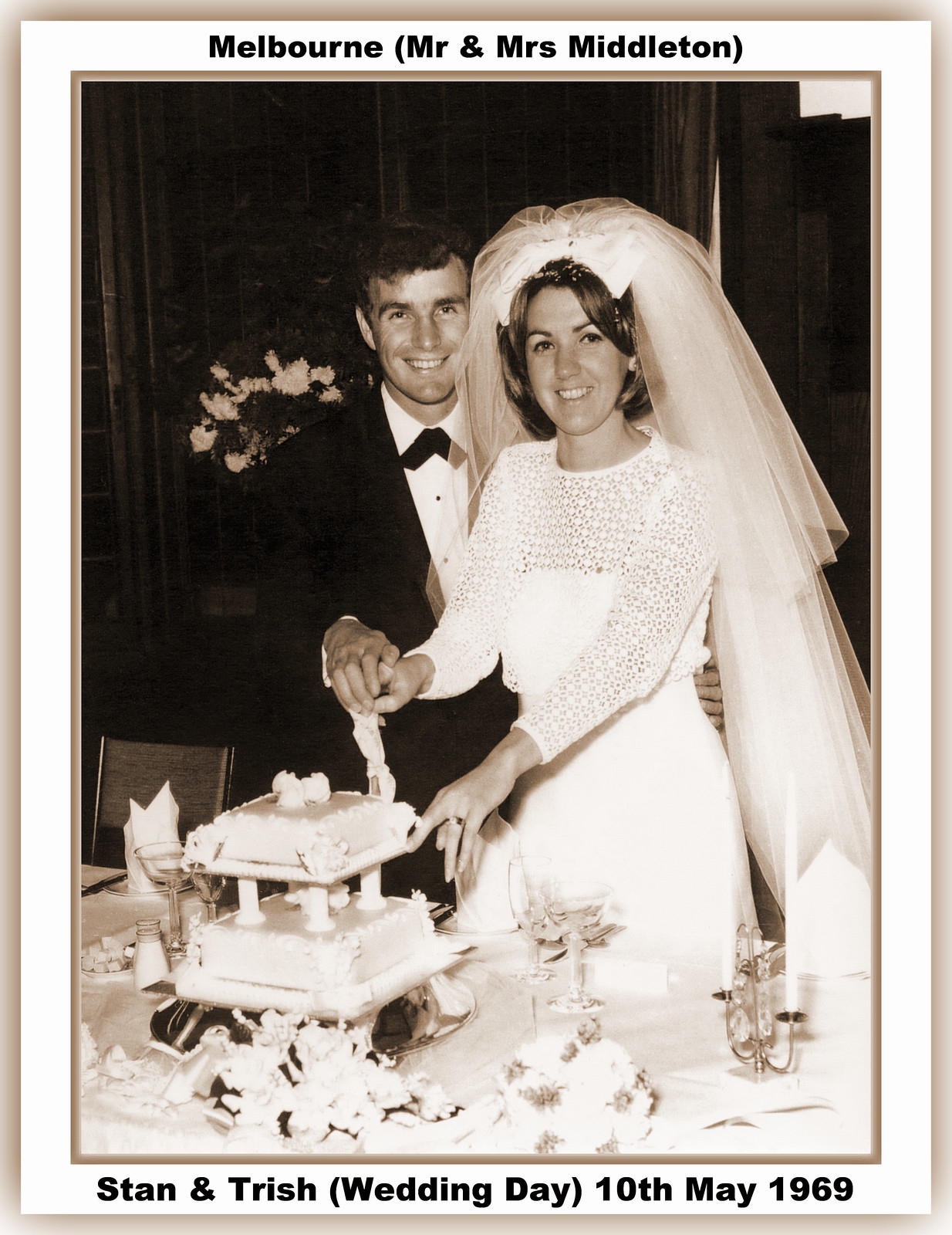This black and white photograph, framed and seemingly aged, captures an intimate moment from the wedding day of Stan and Trish Middleton on the 10th of May, 1969, in Melbourne. The top of the photo bears the inscription "Melbourne, Mr. and Mrs. Middleton," while the bottom reads, "Stan and Trish Wedding Day, 10th May, 1969." The image features the newlywed couple, both with dark hair, standing near a table adorned with flowers, glasses, and possibly a salt shaker. The groom is dressed in a black suit with a white shirt and a bow tie, while the bride wears a long-sleeve, lacy wedding dress and a voluminous veil that flows behind her. They are posed together, hands gently clasped around a knife as they cut into their small, two-layer wedding cake.